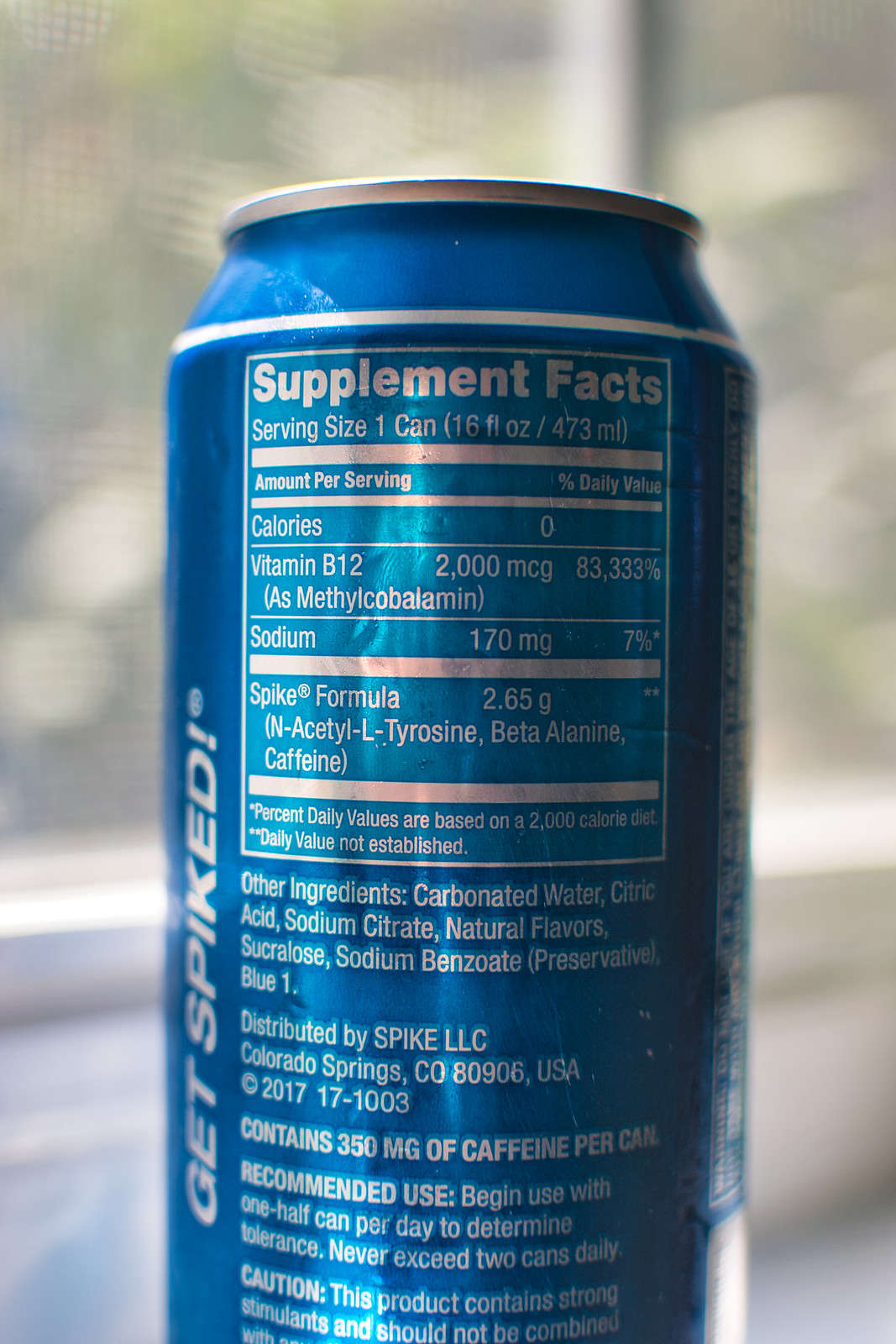This image is a close-up of an energy drink can, prominently featuring its packaging details. The can is predominantly blue with bold white lettering. On the left side, in large, bold capital letters, it reads "GET SPIKED!" with an exclamation mark for emphasis. The main focus of the image is the supplement facts label, providing detailed nutritional information. The serving size is listed as one can, which equals 16 fluid ounces. Notably, the drink contains zero calories and is fortified with an impressive 2,000 mcg of vitamin B12. Additionally, it boasts a proprietary "Spike Formula" totaling 2.65 grams. Visible ingredients include carbonated water, citric acid, and sodium citrate, among others, highlighting the composition of this energizing beverage.